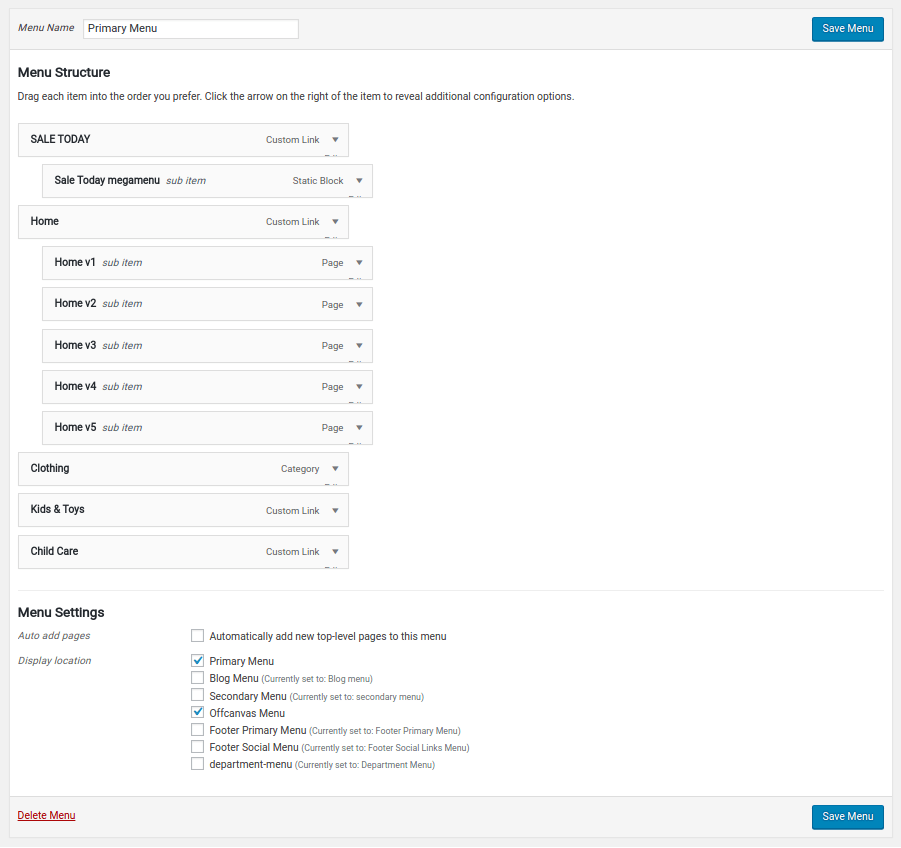Screenshot of Website Settings Menu

The image displays a settings interface for organizing menu options on a website, prominently featuring a mostly white background accented with grey and blue elements for clarity and sectioning. 

**Header and General Layout:**
- The top-left corner exhibits a grey header labeled "Menu Name" above a white box containing the text "Primary Menu".
- In the top-right corner, a blue button with white text reads "Save Menu".

**Menu Structure Section:**
- Below the header, a black title reads "Menu Structure", followed by an instruction in smaller text: "Drag each item into the order you prefer. Click the arrow on the right of the item to reveal additional configuration options."
- A hierarchical menu structure follows, displaying both top-level and nested items:
  - **Sale Today (Custom Link)**: Under this item, nested are:
    - Sale Today, Mega Menu
    - Sub Item: Static Block
  - **Home (Custom Link)**: Nesting beneath this item are:
    - Home V1 (Sub Item, Page)
    - Home V2 (Sub Item, Page)
    - Home V3 (Sub Item, Page)
    - Home V4 (Sub Item, Page)
    - Home V5 (Sub Item, Page)
  - Additional top-level items include:
    - **Clothing (Category)**
    - **Kids and Toys (Custom Link)**
    - **Child Care (Custom Link)**

**Menu Settings Section:**
- Separated by a thin grey line, the "Menu Settings" section includes options like "Auto Add Pages" and "Display Location".
- Accompanying these settings to the right are checkboxes, with options such as "Primary Menu" and "Off-Canvas Menu" marked with blue check marks.
- Other checkbox options listed but not checked include: 
  - Blog Menu
  - Secondary Menu
  - Footer Primary Menu
  - Footer Social Menu
  - Department Menu

**Footer Actions:**
- At the bottom-left corner, red underlined text provides an option to "Delete Menu".
- The bottom-right corner mirrors the save function at the top with a blue button labeled "Save Menu" in white text.

This detailed view encapsulates the settings and structure customization options available for site menus, facilitating an organized and intuitive navigation setup.